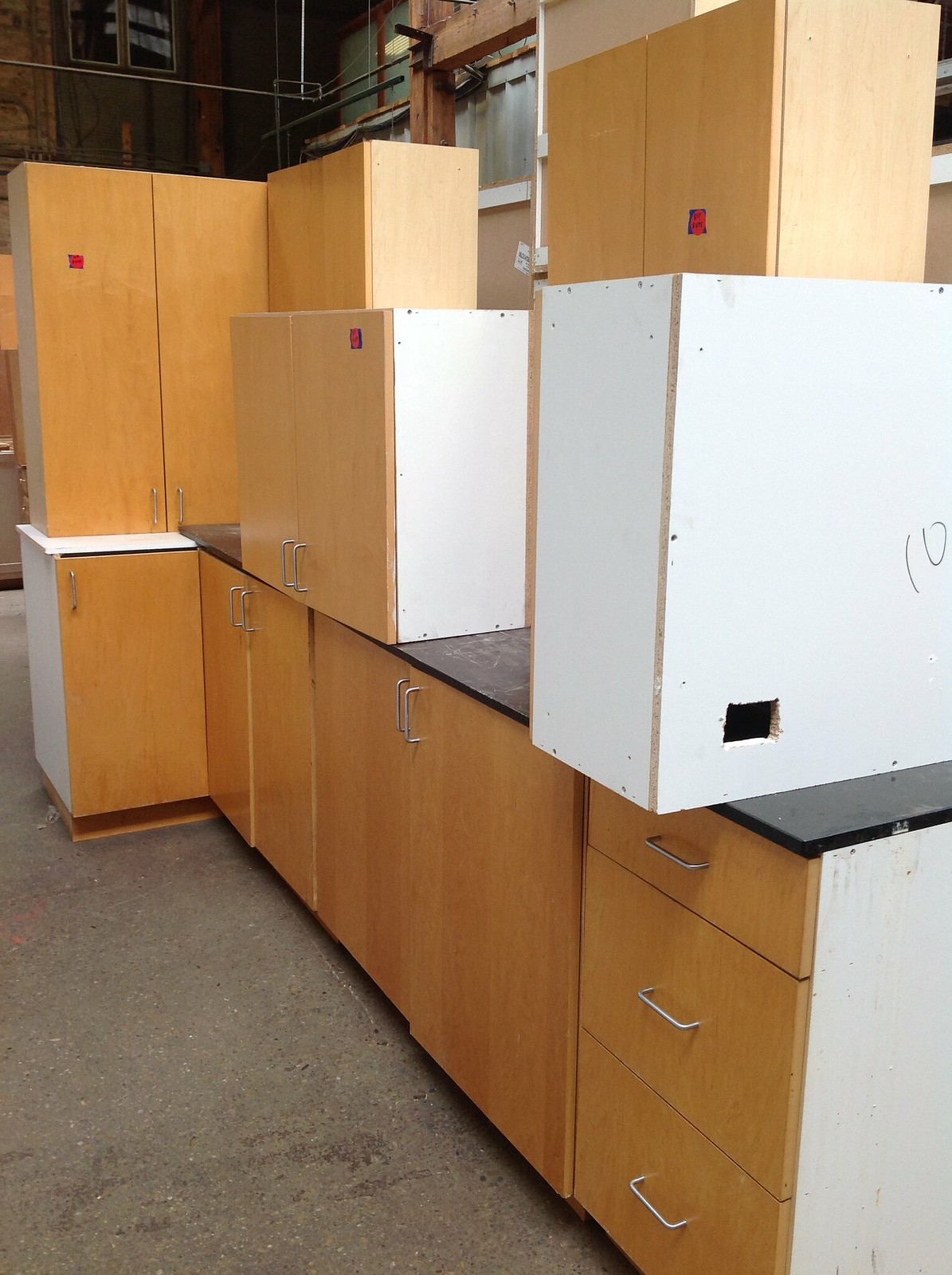The photograph captures a scene inside a warehouse with a concrete floor and overhead piping. Central to the image are a series of wooden cabinets, characterized by their light golden color and metal door handles. These cabinets feature black countertops and white side panels. There are additional stacked cabinets, which give the appearance of a display setup or construction area. Specifically, on the bottom left, there are three horizontal drawers with gray handles next to two vertical cabinets, also with gray handles. In the bottom right corner, a white outer edge of the cabinets is visible. Two additional cabinets are seated atop these, one predominantly white and another showing both its white side and light wooden brown front. The background includes another set of cabinets and visible black ceiling pipes, adding to the industrial ambiance of the scene.